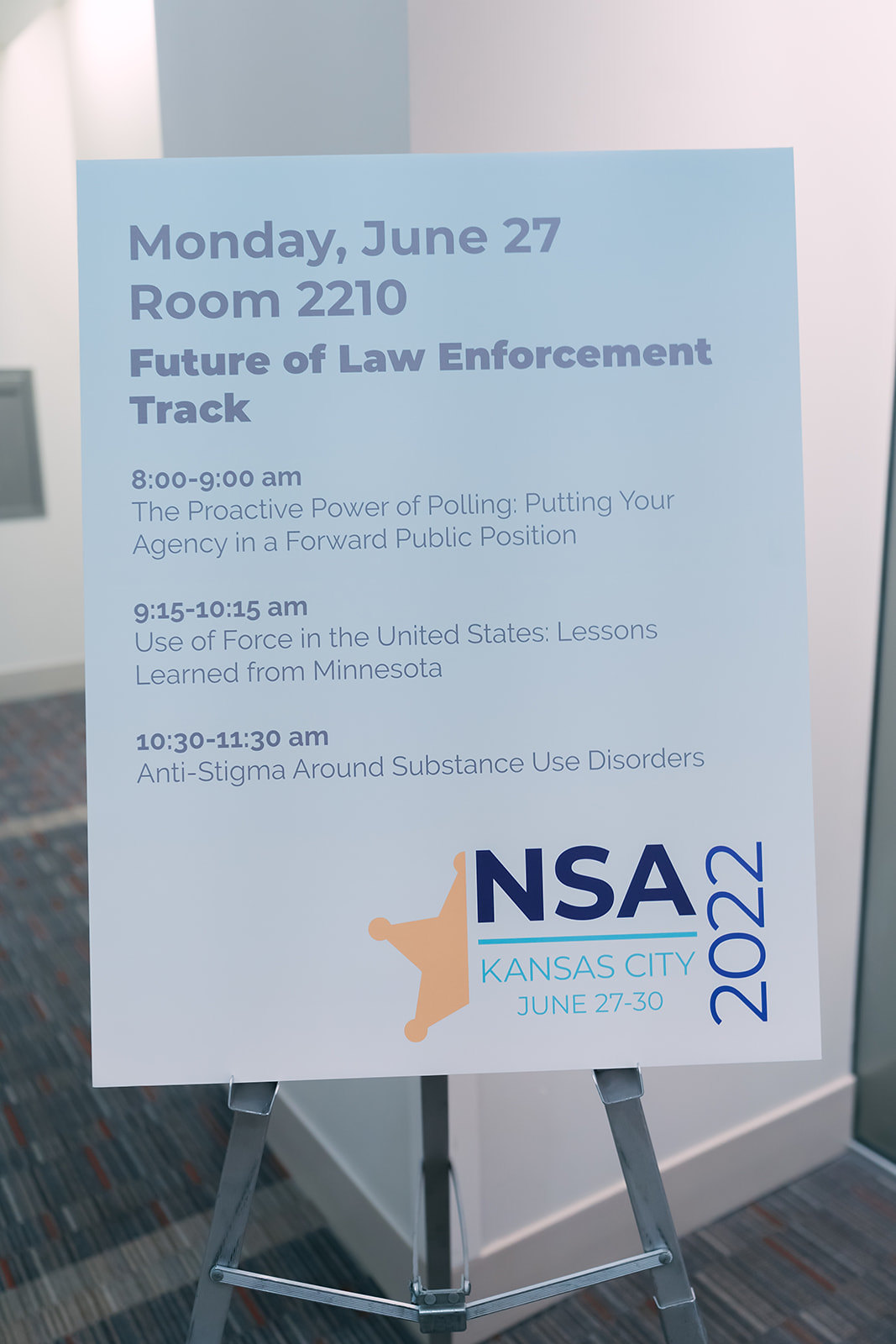The image features a large poster board on a partially visible steel easel. The poster, predominantly white with black text, details the schedule for the "Future of Law Enforcement Track" on Monday, June 27, in room 2210. The events listed include:

- 8:00 to 9:00 a.m.: "The Proactive Power of Polling, Putting Your Agency in a Forward Public Position"
- 9:15 to 10:15 a.m.: "Use of Force in the United States, Lessons Learned from Minnesota"
- 10:30 to 11:30 a.m.: "Anti-Stigma Around Substance Use Disorder"

At the bottom right of the poster, there's the logo of the NSA conference in Kansas City, happening from June 27 to 30, 2022. The logo includes a partially cropped golden sheriff's badge, displaying only three points and the year 2022 positioned vertically. The background shows a convention hall setting with mixed red, blue, and gray carpeting, a white wall with cream-colored baseboards, suggesting a hotel venue.